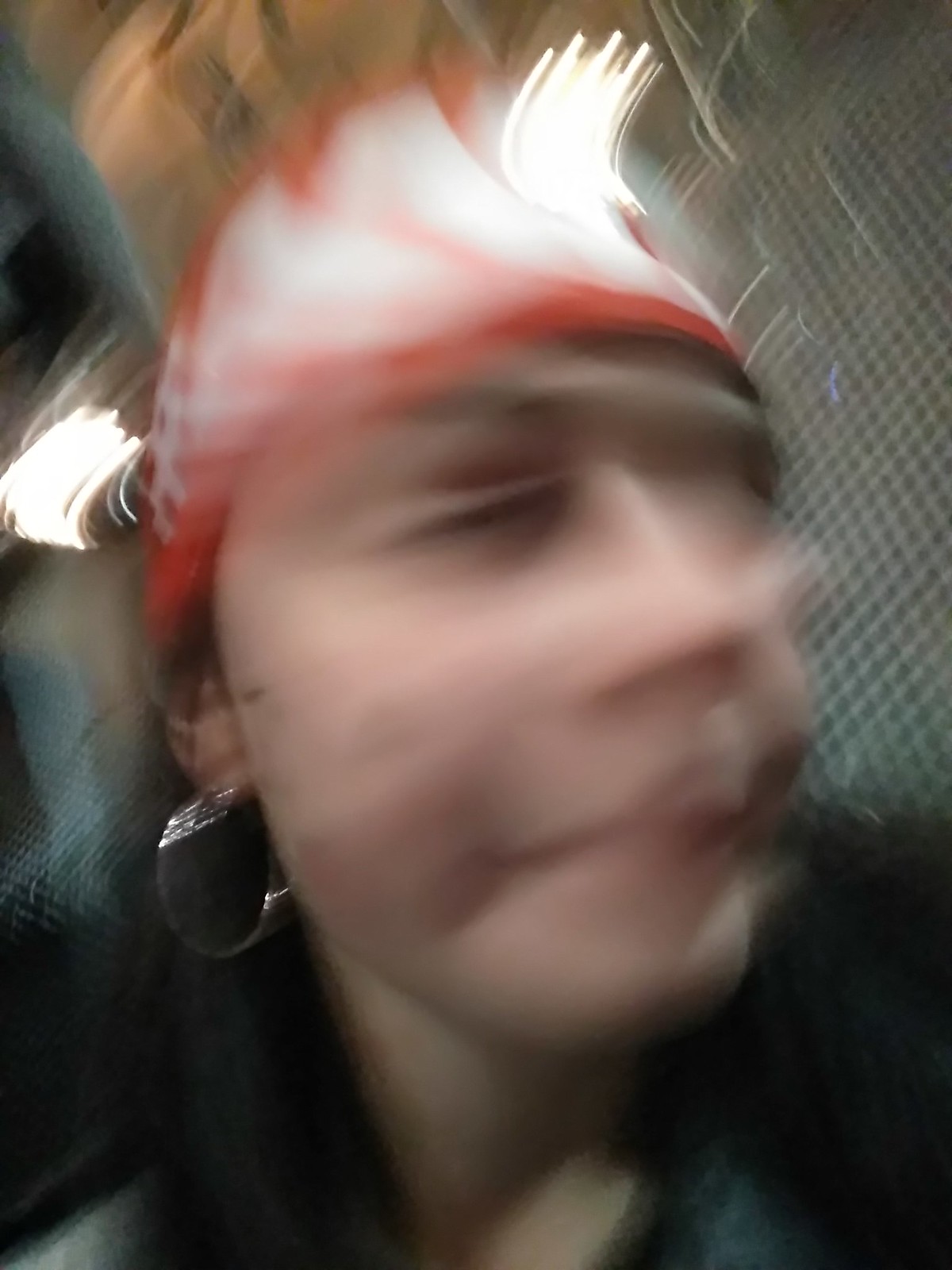The image depicts a blurred face of an individual with an indifferent expression, exuding a nostalgic yearning for the "good old days" when their mother sang them to sleep, contrasting with their current feeling of being stressed out. They are adorned with a silver earring and a red bandana or headscarf, along with an assortment of indistinguishable items on their head, including a hat, helmet, paper, or napkin, contributing to a chaotic appearance. The top of their head is obscured by a large white blur, flanked by additional blurs in white, brown, and orange hues. The right side of the image is characterized by a checkered pattern blur. Below the face, a neck is visible. The sides of the neck are bordered by black blurs, transitioning into gray blurs immediately below, creating a layered effect of indistinct colors and patterns.